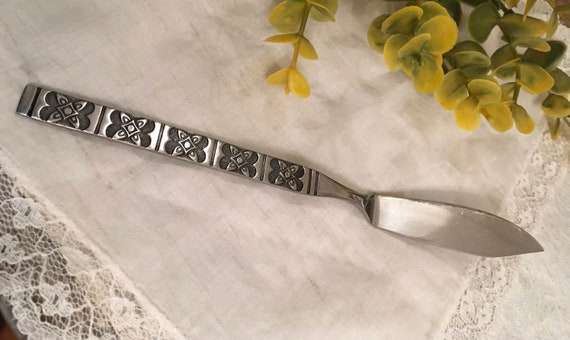In this photorealistic image, an old-fashioned specialty knife lies horizontally on a white lace tablecloth, which has embroidered lace edges visible on both the left and right sides. The knife, with its silver metallic finish, features a long handle embellished with five X-shaped abstract flower designs, each separated by black lines. The handle, slightly elevated on the left side, curves downward toward the blade, which is positioned lower on the right side of the image. The blade itself resembles that of a butter knife but is sharper, possibly intended for serving soft cheeses. In the upper right corner of the image, branches of a green plastic plant with small oval-shaped leaves drape slightly over the white cloth, adding a touch of color to the scene.